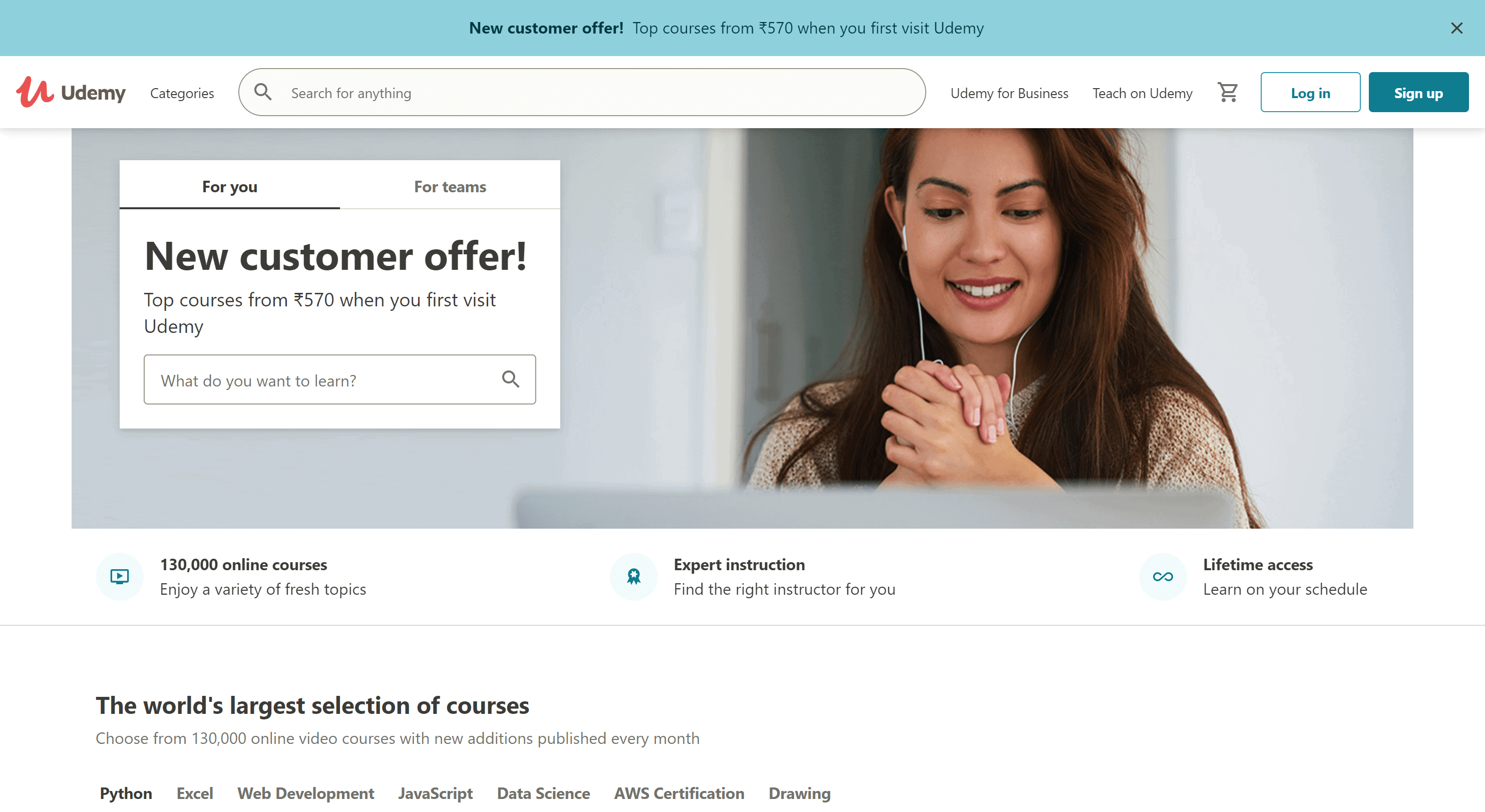The image showcases the Udemy website, featuring a predominantly gray and white color scheme with a teal accent at the top. A promotional banner highlights a new customer offer with top courses available for 570 rubles. The website caters to both individual users and teams, emphasizing its extensive catalog of 130,000 online courses, expert instruction, and lifetime access. Prominent course categories include Python, Excel, web development, JavaScript, data science, AWS certification, and drawing.

In the foreground, a smiling olive-skinned woman with dark hair is depicted wearing earbuds. Seated in front of a laptop, she appears to be engaged in an online course. She is dressed in a beige top or sweater, enhancing the image's warm and inviting atmosphere.